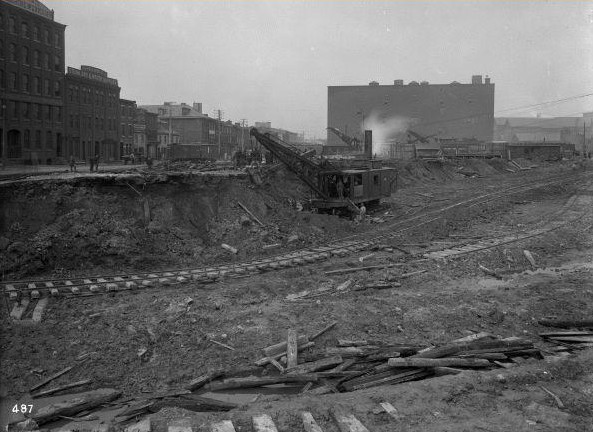This black-and-white photograph, marked "487" in white font at the bottom left, appears to document a construction site or a demolished urban area. The foreground is dominated by torn-up railroad tracks, with wooden planks scattered and piled haphazardly, indicating recent upheaval. A large piece of construction equipment or a crane is visible towards the center of the image, suggesting ongoing work. The background reveals a mix of old and tall buildings, possibly indicative of an urban environment undergoing redevelopment or desolation. Furthermore, a few distant figures can be seen near the buildings, adding a sense of scale to the scene. The sky appears dark but without clouds, contributing to the somber tone of the image.